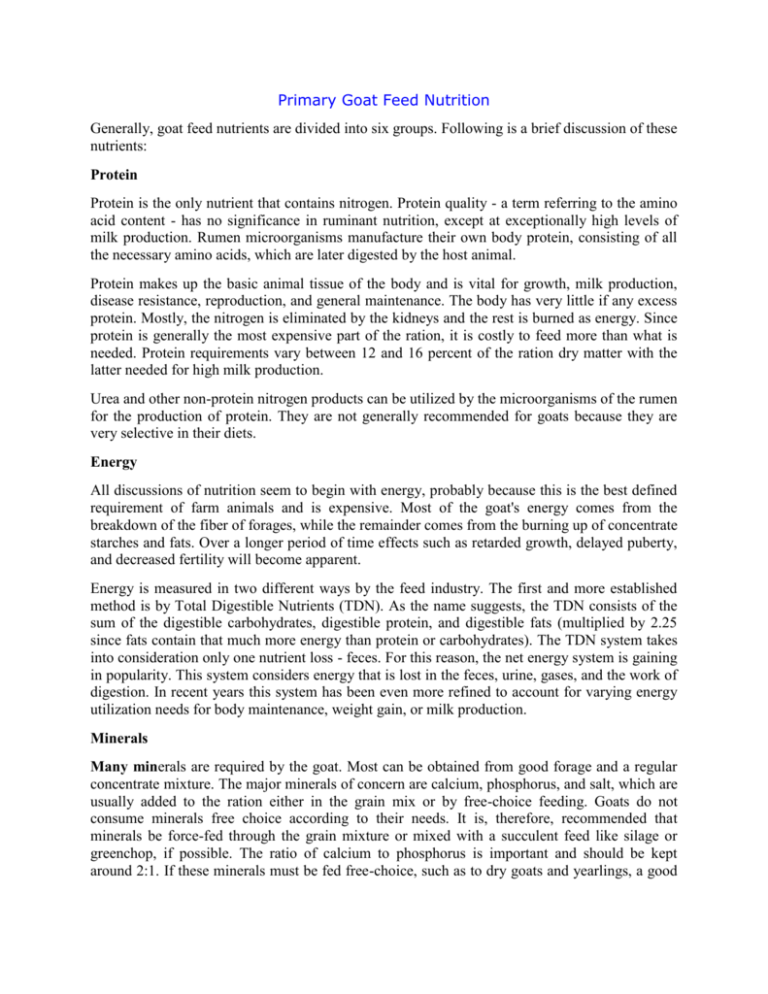The image features a document titled "Primary Goat Feed Nutrition," with this title prominently displayed in blue at the center. Below the title, the document is organized into multiple paragraphs that detail key nutritional components critical for goat feed. 

The first paragraph provides an overview, stating that goat feed nutrition is categorized into six primary groups, followed by a brief discussion of each nutrient. 

The discussion begins with the first group, **Protein**, which is highlighted in bold black font. The text emphasizes that protein is the only nutrient containing nitrogen and mentions the concept of protein quality, which refers to amino acid content. It explains that protein quality has minimal significance for ruminant nutrition, and continues with further details in two additional paragraphs.

Next is the section on **Energy**, which spans two paragraphs. It underscores that all discussions on nutrition should start with energy, given it is the most precisely defined requirement for farm animals and also one of the most expensive nutrients to provide.

The final section covered in the visible portion of the document is **Minerals**. This section consists of one paragraph. However, the last sentence appears to be cut off, suggesting that more text follows beyond what is shown in the image.